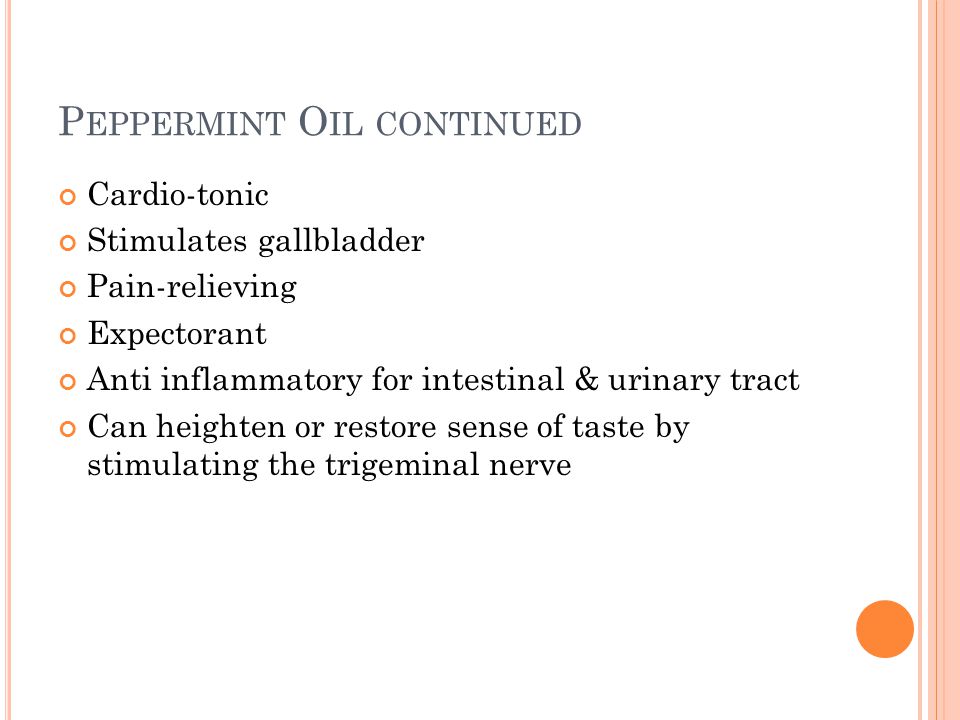The image is a PowerPoint slide titled "Peppermint Oil Continued" in dark gray letters at the top left. The text is left-aligned and presented on a white background with six black text bullet points, each marked by an open circle. These bullet points detail the benefits of peppermint oil: 1) Cardiotonic, 2) Stimulates Gallbladder, 3) Pain Relieving, 4) Expectorant, 5) Anti-Inflammatory for Intestinal and Urinary Tract, and 6) Can Heighten or Restore Sense of Taste by Stimulating the Trigeminal Nerve. The slide features a thin pink vertical stripe on both the left and right sides, with an additional thicker rectangular pink border on the far right. An orange circle is positioned at the bottom right corner of the slide.